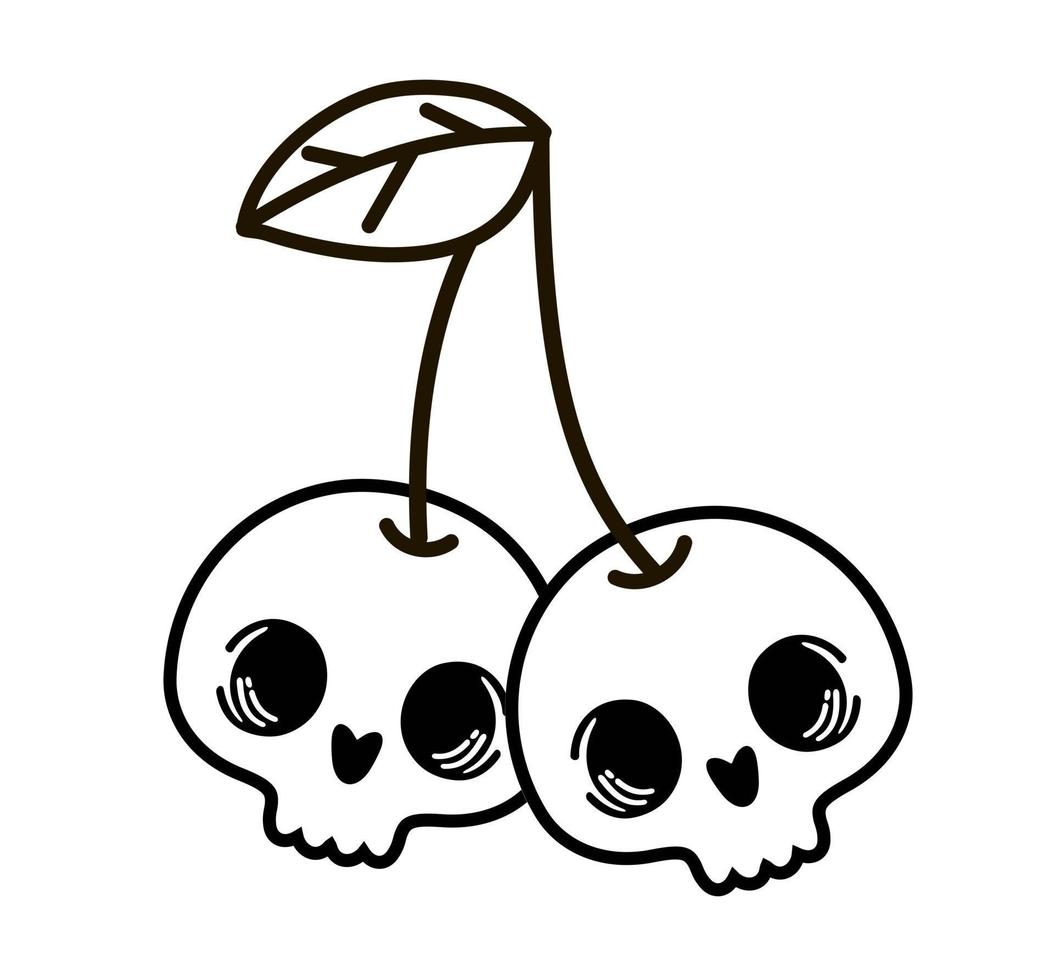This black and white illustration creatively transforms the imagery of cherries into a pair of cartoony skulls. Each skull features large, sunken eyes, a heart-shaped nose, and four front teeth, devoid of jaws. The skulls imitate the round shape of cherries, connected to two stems that converge on an ovate leaf with detailed veining. The skulls are arranged with one slightly behind the other, enhancing the depth of the artwork. Drawn entirely in black lines with white highlights for the skull faces and the leaf, this monochromatic sketch delivers a playful yet eerie visual twist on the familiar fruit.